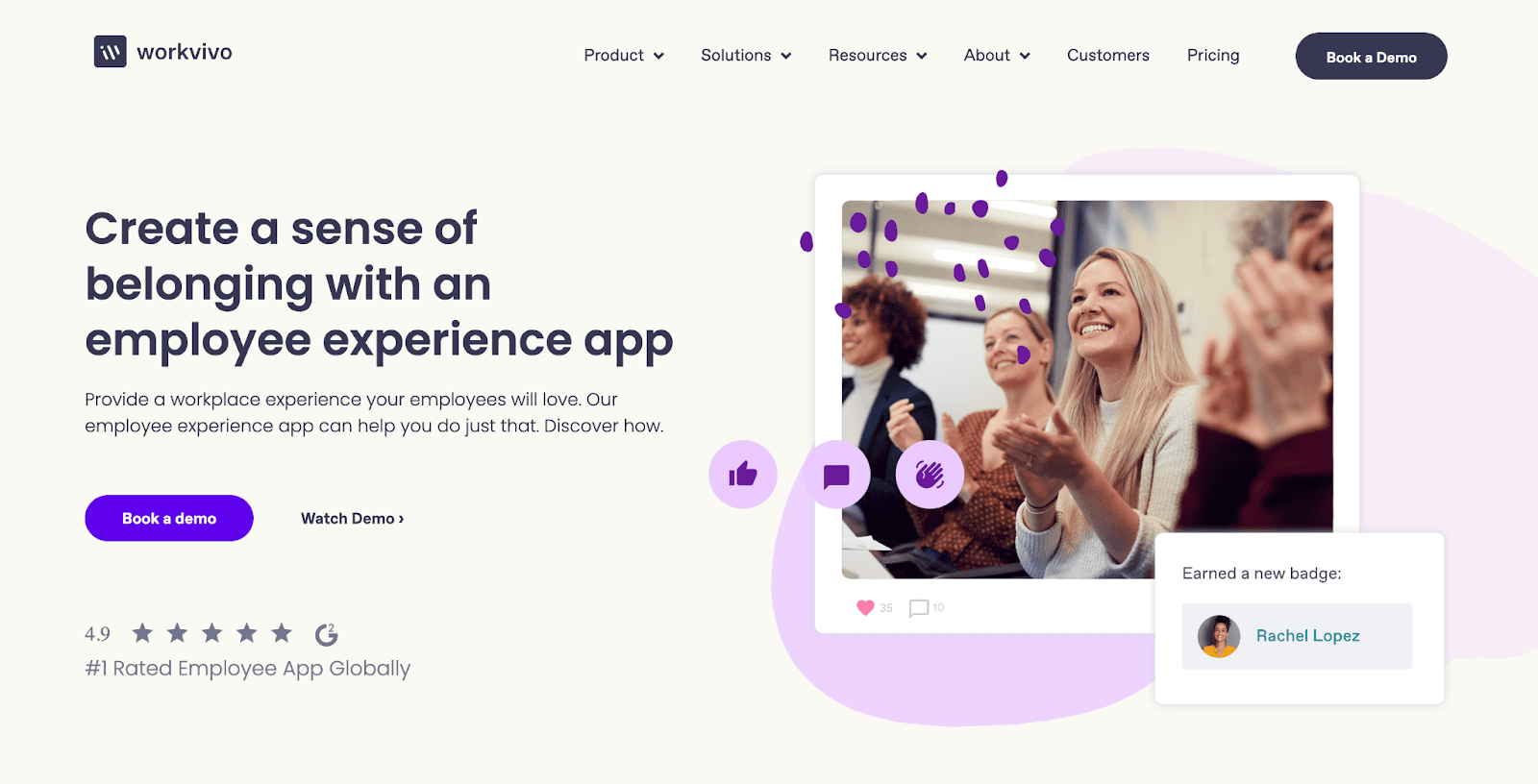The upper left corner of the image displays the logo "VIVO." Positioned in the top right, starting from the center, are a series of labeled menu items: "Product" with a downward menu, "Solutions" with a dropdown menu, "Resources" with a dropdown, "About" with a dropdown, "Customers," "Pricing," and a prominent black button with white text that reads "Book a Demo." 

Along the left side of the image, there is a call to action: "Create a sense of belonging with an employee experience app. Provide a workplace experience your employees will love. Our employee experience app can help you do just that, discover how." Below this text is a purple button labeled "Book a Demo" in white font, followed by a button that reads "Watch Demo" with a right arrow.

The image further highlights a 4.9-star rating from G2 and mentions that it is the "#1 rated employee app globally." 

In the center of the image is a graphic resembling a Polaroid photo, depicting a group of women who are seated, clapping, and smiling. Above the photo are three interactive icons: a thumbs up, a comment bubble, and a wave. Below the photo are a red heart and a comment count, indicating "35 loves" and "10 comments." Lastly, the image includes a message stating, "Earn a new badge, Rachel Lopez," all set against a background featuring shades of purple, black, white, and gray.